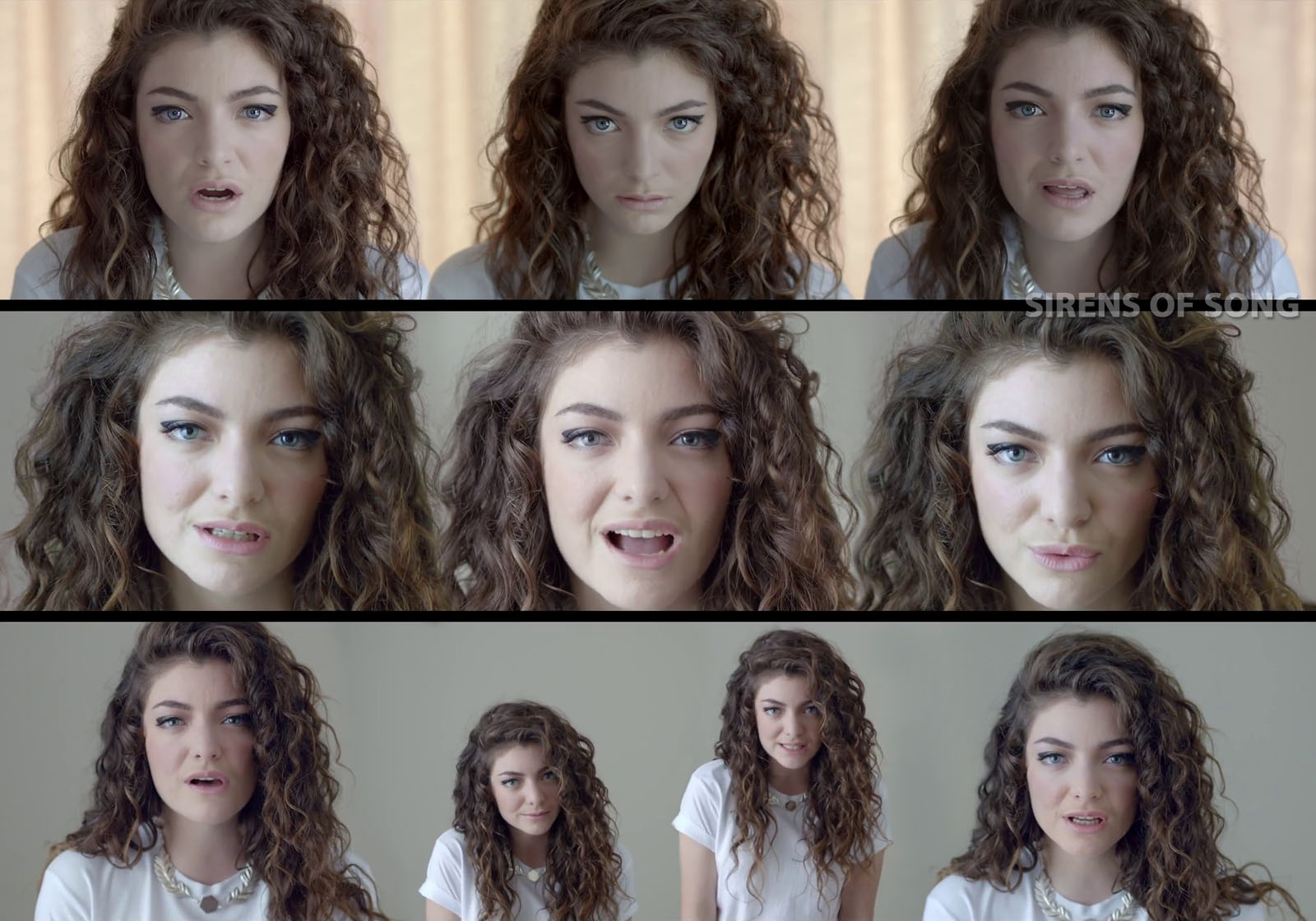The image features a series of screen caps from a music video by the singer Lorde. There are three distinct strips of photos stacked vertically and centered, creating a neatly organized and easy-to-view composition. Each strip showcases a different perspective of Lorde with the top strip featuring a pinkish background, and the bottom two strips having grayish ones. The images predominantly display Lorde's face, captured multiple times, totaling approximately ten repeated shots.

In the photos, Lorde is gazing intently into the camera, her hair styled with long curls cascading past her shoulders and a section combed to one side. She is dressed in a black t-shirt and adorned with a laurel-wreath-styled necklace with a coin pendant. The tiers of images are separated by black stripes, with the top tier consisting of three pictures, the middle tier focusing more closely on her face with three images, and the bottom tier showing four pictures taken from a slightly greater distance. The image also contains a watermark on the right side that reads "Sirens of Song." 

The colors present in the image include a palette of pink, brown, tan, blue, white, and gray, which together create a cohesive visual aesthetic.